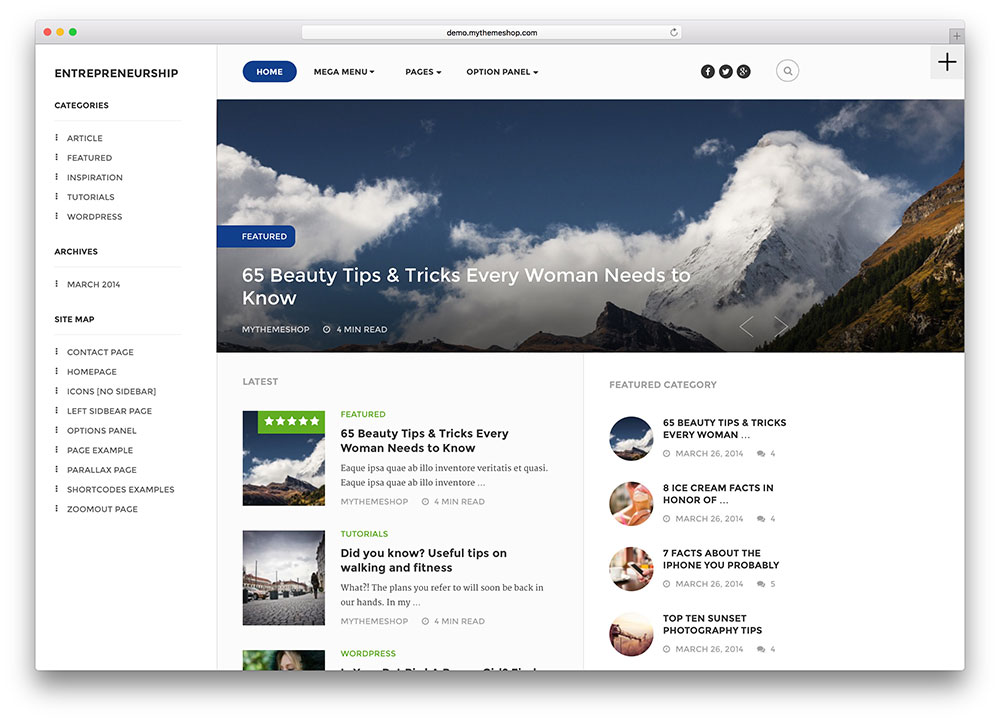The image depicts a screenshot taken from an Apple Mac computer, evident by the distinctive red, yellow, and green dots located at the top left corner of the browser window. At the center, the browser URL bar displays the website address "demo.mythemeshot.com," accompanied by a refresh button to its right and, further to the right, a plus sign for opening new tabs.

The website itself features a vertical navigation box on the left side, titled "ENTREPRENEURSHIP" in bold, uppercase black letters beneath the tri-colored dots. This box contains various categories in smaller, capitalized text: Articles, Features (each on a separate line), Inspiration, Tutorials, and WordPress. Below these categories, the Archives section lists "March 2014," and a bolded "SITEMAP" header is followed by links to pages such as Contact, Home, Icons, Left Sidebar Page, Options Panel, Page Example, Parallax, Parallax Page, Shortcuts Example, and Zoom Out Page.

At the top center of the webpage, a horizontal navigation menu spans from left to right, starting with "Home" highlighted in blue within an oval shape, indicating the current selection. This is followed by "Mega Menu" with a dropdown option for various pages and an Options Panel also featuring a dropdown box. 

Prominently displayed beneath this navigation bar is a featured article titled "65 Beauty Tips and Tricks Every Woman Needs to Know," accompanied by an image of serene mountains enveloped in clouds with rocky terrain. The section titled "Latest" showcases three columns each featuring different images linked to articles, categorized under Features, Tutorials, and WordPress. Overall, the webpage also includes a Featured Category section and four additional articles along with comment sections for user engagement.